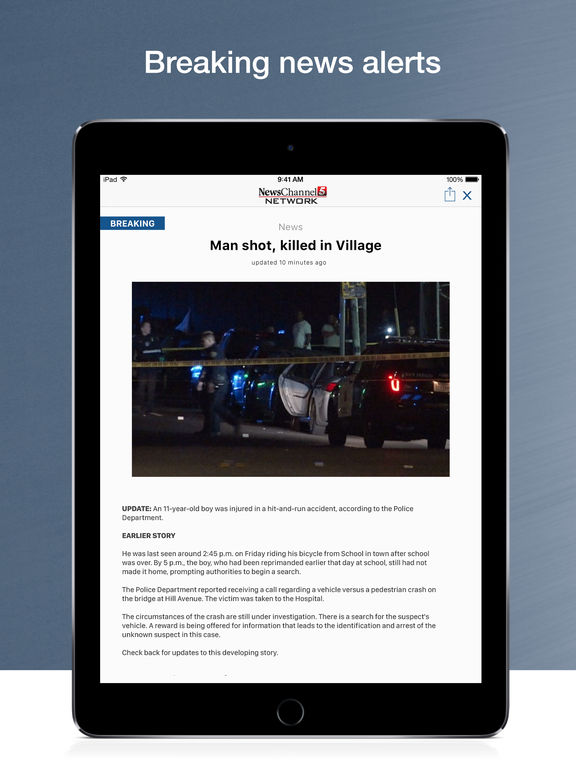The image captures a mobile phone with a black exterior and a white screen displaying a news article from News Channel 5 Network. The background of the image includes a bold "Breaking News Alert" banner in white on a red rectangle. The headline on the phone reads, "Breaking: Man Shot and Killed in Village," with an update timestamp of 10 minutes ago. Below the headline, a yellow crime scene tape adorned with "Do Not Cross" text is visible, adding to the gravity of the news.

In the image, several police cars and officers are seen, alongside bystanders observing the scene. The article continues with an additional update: "An 11-year-old boy was injured in a hit and run accident, according to the police department." The earlier part of the story details that the boy, who was last seen around 2:45 p.m. on Friday riding his bicycle home from school, had not returned by 5 p.m., leading authorities to initiate a search. The circumstances are still being investigated, and the article urges readers to check back for further updates on this developing story.